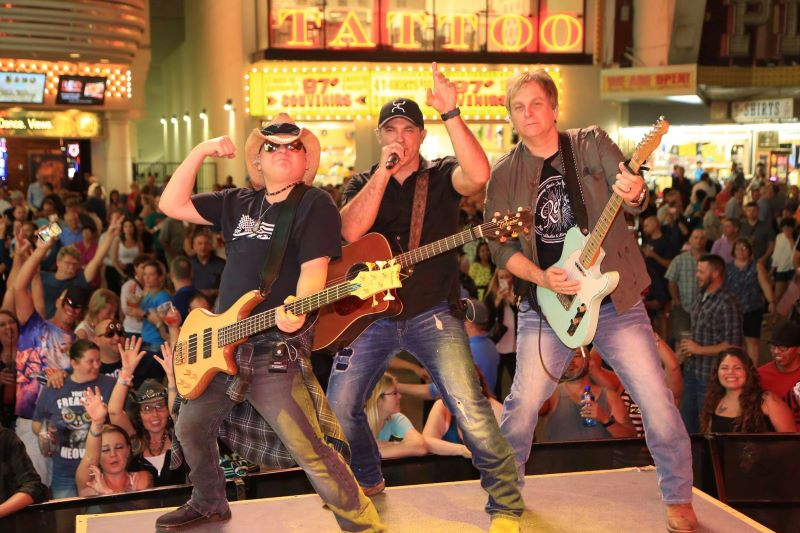The image captures an outdoor concert set in a vibrant cityscape at nighttime, with bright lights and multiple signs in the background, including a prominent "Tattoo" sign. On stage, three older male musicians are playing guitars and singing. The performers, all wearing jeans, include one wearing a white cowboy hat and sunglasses, one in a black baseball hat singing into a microphone, and the third with an open shirt and no hat. Their guitars vary in color: yellow electric, brown acoustic, and blue electric. Behind them, a lively crowd is visible, enjoying the performance with smiles, raised hands, and phones. The scene is filled with a mix of faded blue-green, mahogany, beige, and neon colors, contributing to the energetic, festive ambiance of this outdoor venue.